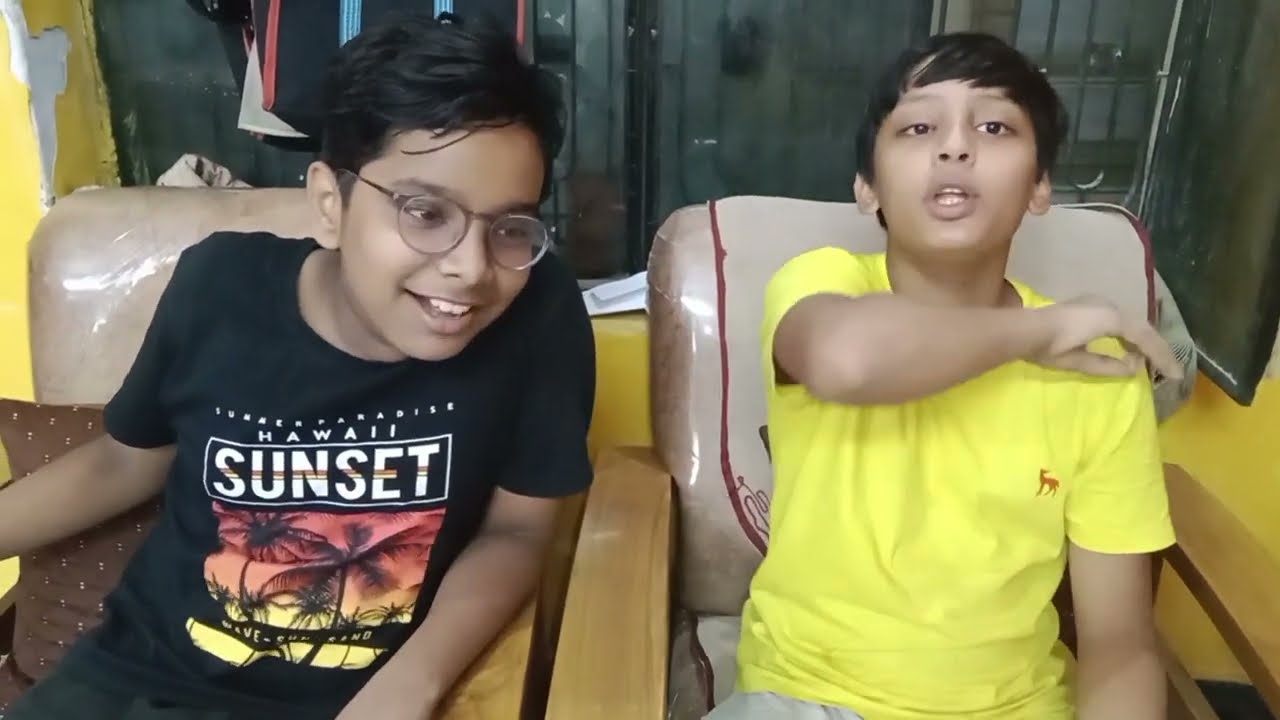In the photograph, two Indian boys are seated in identical wooden chairs with beige cushions. The boy on the left is wearing glasses and has black hair and brownish skin. He is dressed in a black t-shirt featuring a "Hawaii Sunset" graphic, depicting palm trees and a tropical sunset. He leans slightly forward, looking downwards around the 5 o'clock position, and is smiling. The boy on the right, also with black hair and olive skin, is wearing a yellow shirt with a small deer symbol and gray pants. His right arm is raised, with his elbow bent and his hand near his left shoulder. His lips are pursed as if he is speaking. The boys are positioned in a room with yellow walls, some parts chipped away, and a window featuring black sheer curtains and metal bars. The setting behind them includes a light black backdrop, contributing to a somewhat nondescript environment.